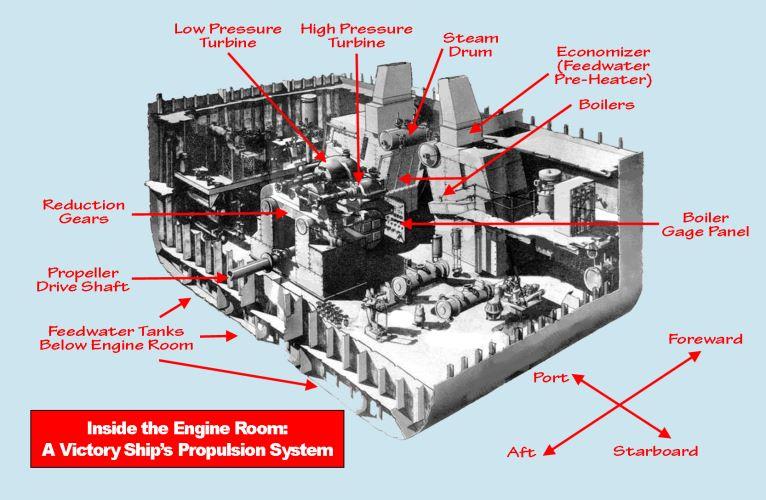This detailed diagram, set against a pale blue background, illustrates the intricate propulsion system inside a Victory ship's engine room. Centrally, the diagram features a large grayscale etching of the engine, surrounded by numerous red arrows and labels highlighting its many components. At the bottom left, a red rectangle with white text reads "Inside the Engine Room: A Victory Ship's Propulsion System." 

The cutaway reveals various machinery parts, starting with feed water tanks below the engine room, identified by three corresponding arrows. Above these are the propeller drive shaft and reduction gears. The top section of the diagram highlights the low pressure turbine, high pressure turbine, steam drum, economizer (feed water preheater), and boilers. 

To the right side, the boiler gauge panel is indicated. Additionally, a compass-like orientation symbol near the red callout box denotes the directions: forward, starboard, aft, and port. The entire layout, densely packed with mechanical details, provides a clear and comprehensive view of the steam-driven engine that propels the ship, with essential components like turbines, reduction gears, and feed water systems all meticulously labeled.